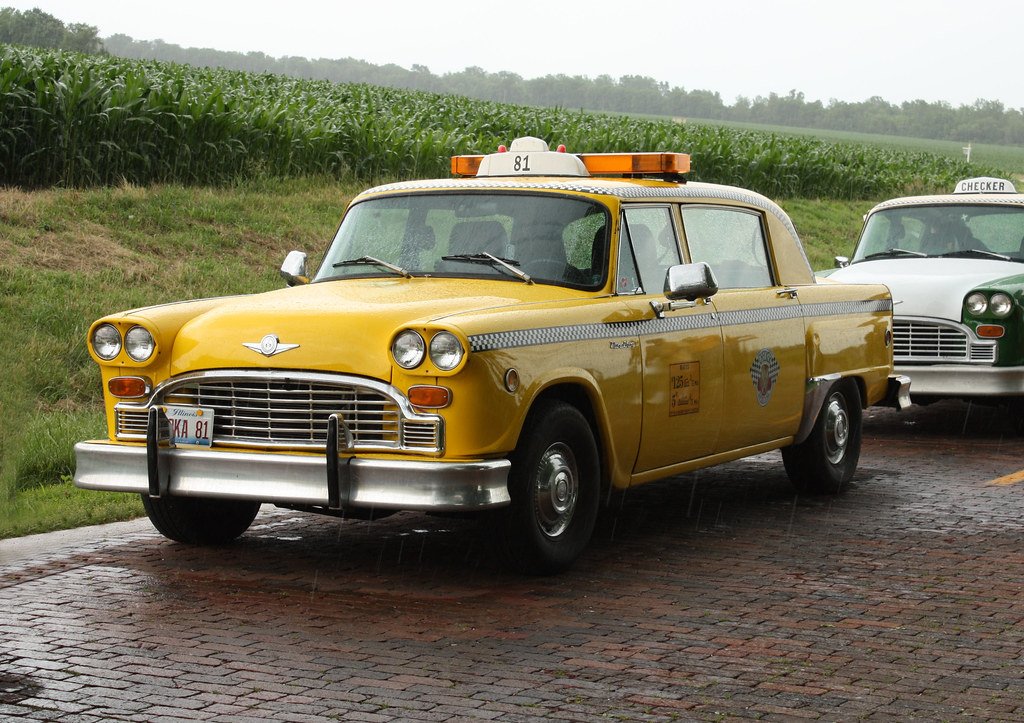This photograph captures a vibrant scene featuring two vintage taxis parked on a distinctive red brick driveway, which appears wet from a recent rain. The focal point is a bright yellow taxi from the 1960s or early 70s, numbered 81, adorned with a checker pattern along its sides and sporting a white license plate with red lettering and a blue bottom. Positioned slightly behind and to the right of the yellow taxi is another classic checker cab, this one predominantly green with a white hood, and clearly marked "Checker" on its top. Both vehicles are stationary in front of a lush backdrop comprising a row of tall corn plants and a dense tree line, with no buildings or people in sight, emphasizing their solitary presence in this serene, somewhat rural setting.